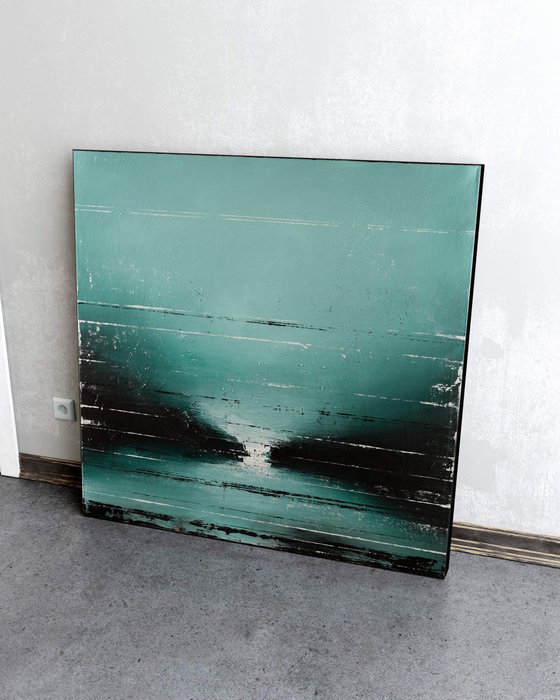In this color photograph, a square abstract painting leans against a white wall with gray baseboards, situated on a gray tile floor bordered by brown trim. The composition of the painting is complex and distressed, featuring a blurry landscape that melds into abstract shapes. Dominated by hues of bluish-green and aqua, the painting is accented with sporadic black areas that resemble wide-mouthed Vs toward the bottom corners. White brush strokes traverse the canvas, creating a connection between a large hourglass-shaped figure at the top and a smaller, shallow one at the bottom. Additional thin horizontal stripes in black and white add to the textured layers of the artwork, evoking an impression of fragmented, tapering land masses converging towards a shared horizon.